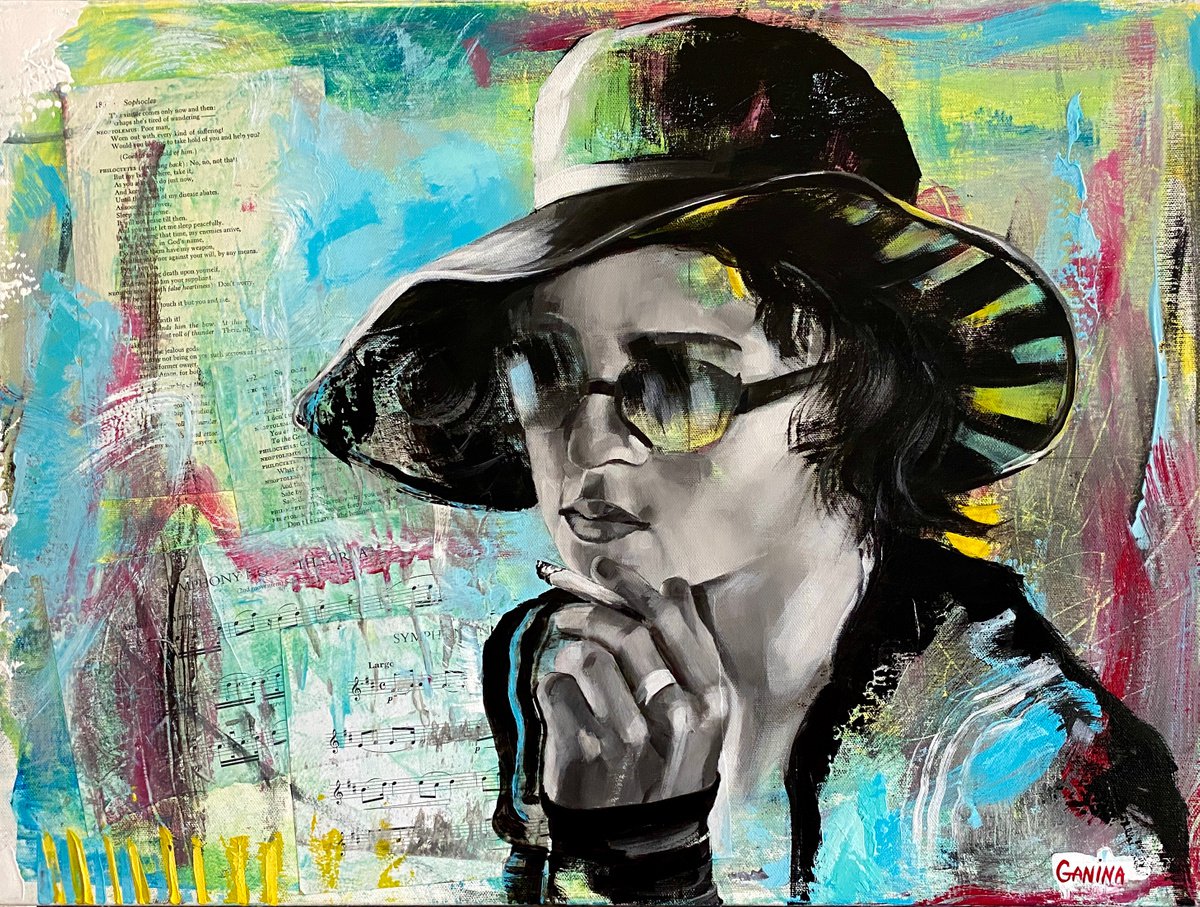The image is a vibrant mixed media artwork likely created digitally, showcasing a young woman in her late 20s. The background is an eclectic collage of pages from books and musical notation, all splashed with an array of vivid colors including blue, green, red, purple, yellow, pink, gold, and brown. In the foreground, the woman is rendered mainly in black and white, with touches of color. She wears a distinctive black sun hat with yellow-green streaks under the brim and a small green spot on top. Her sunglasses are uniquely colored, with the lens on the left featuring a yellow or orange tint, and the lens on the right exhibiting a blue hue. She sports a black shirt accentuated by blue, white, and gray stripes. Her pose is dynamic, facing slightly to the left while holding a cigarette between her pointer and middle fingers, with a noticeable ring on her middle finger. Her expressive face is framed by dark lipstick, and she seems lost in thought, touching her chin gently with her left hand. The backdrop features artistic scenery, possibly depicting skies and Southwestern landscapes, which further enriches the vivid and layered composition of the artwork.